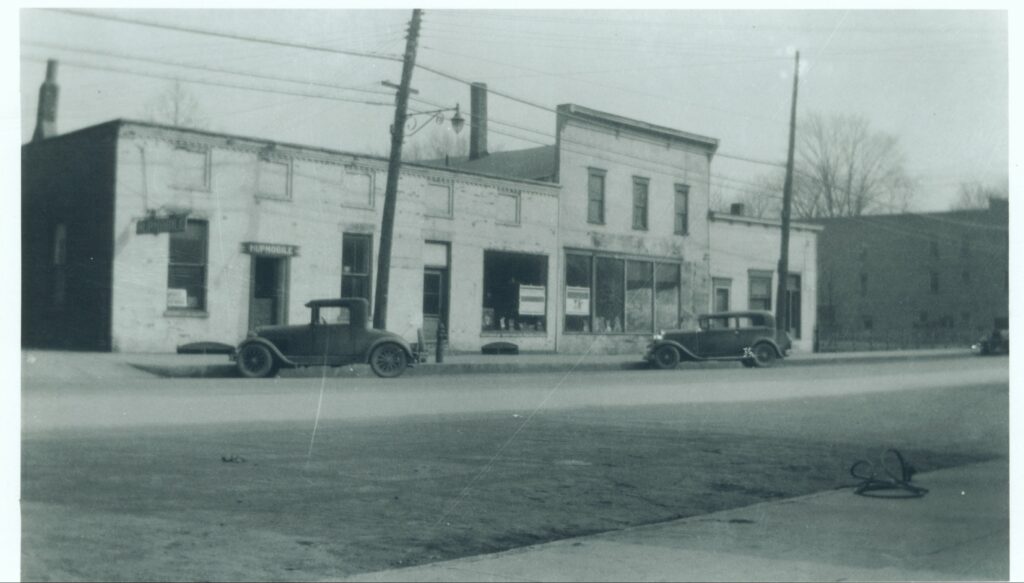This vintage black-and-white photograph, likely from the 1920s or 1930s, depicts a bustling street scene featuring two old-style cars—the first a two-door coupe and the second a four-door sedan—parked along a dirt road that looks compacted and smooth. The cars are stationed in front of a row of four buildings, each appearing to be businesses with noticeable storefronts. Two of the buildings have small windows, while one features a longer storefront window. Above the parked cars, several telephone poles can be seen with lines extending from them, indicative of the era's infrastructure. Off to the right in the distance, the photo also captures another building along with what appears to be some trees under an overcast sky. The overall ambiance of the scene is one of an old and perhaps somewhat run-down street, deeply characteristic of its time.